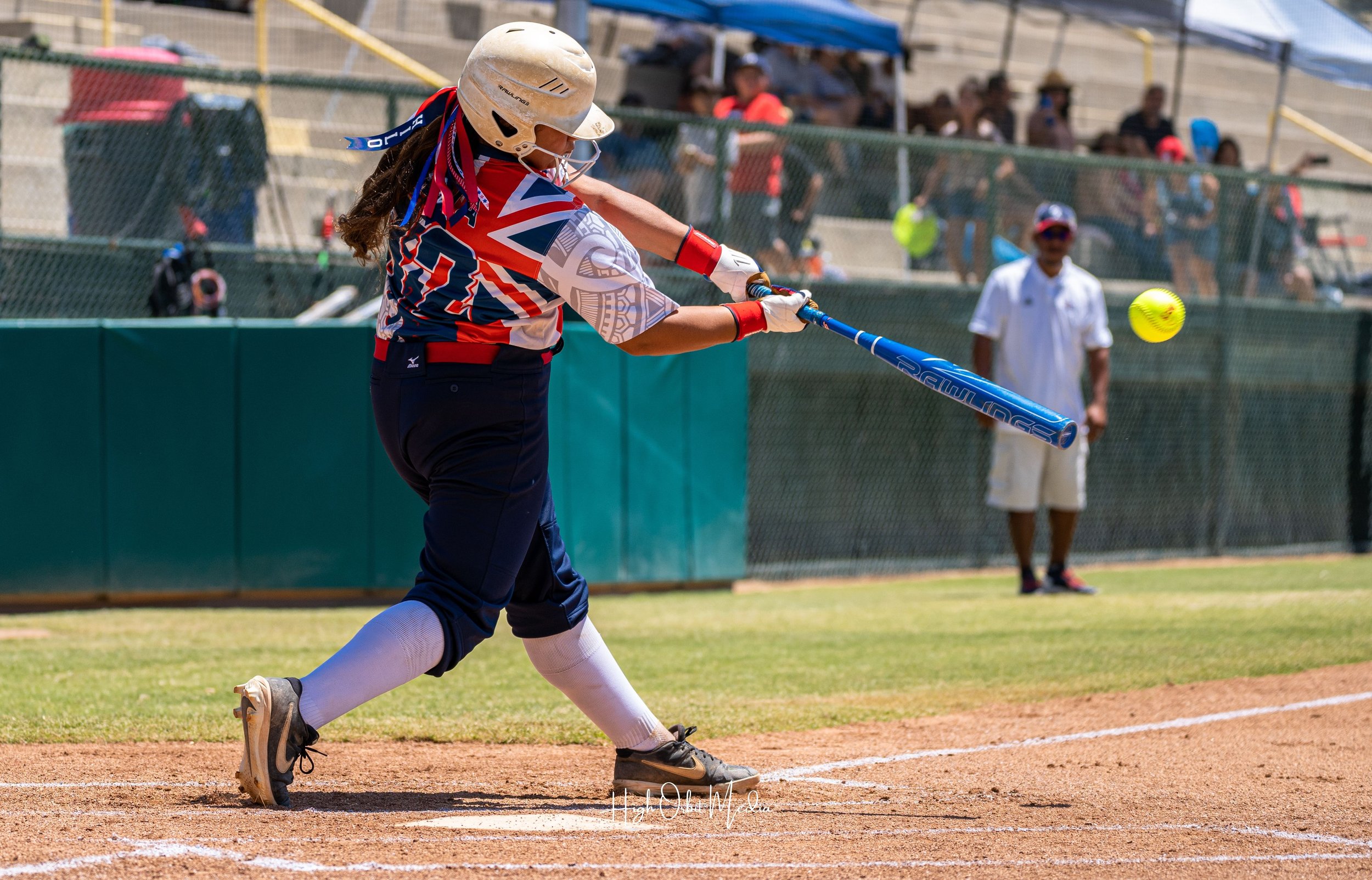The vibrant full-color photograph captures a dynamic moment in a baseball game on a sunny day. A young girl, identifiable by her dark skin and long dark hair, is poised mid-swing as she aims to hit a yellow baseball with her blue metal bat. She is fully geared up, wearing a white batting helmet with a face mask, gloves, and a patriotic red, white, and blue short-sleeved jersey emblazoned with the British Union Jack and the number 2 on her back. Her uniform is completed with navy blue knee-length pants, white knee socks, and black tennis shoes featuring yellow stripes, likely Nike. The sun illuminates the field, highlighting the sparse audience seated behind the fence in the bleachers, and a man, possibly a coach or umpire, standing in the middle right of the frame in a white shirt and beige shorts. Overall, the image conveys the intensity and focus of a lively baseball match.